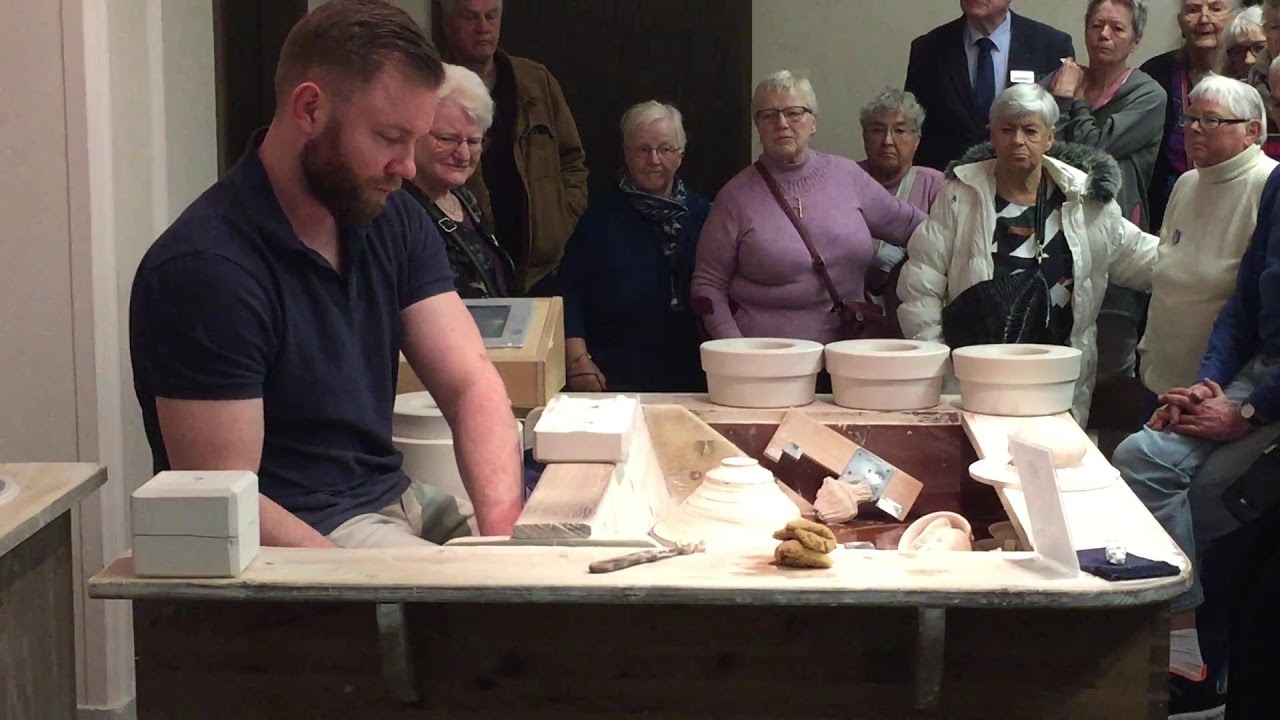The photo captures a young Caucasian man with short brown hair and a neatly trimmed beard and mustache, clad in a black short-sleeved collared shirt and light tan khaki pants. He is seated at a wooden workstation adorned with a variety of tan clay pots. The setting appears to be indoors. The man, who is engrossed in his task, is demonstrating pottery-making techniques. This includes turning the clay, which is evident from the two six-by-six-inch blocks of clay placed beside him. Although his hands are obscured by the ledge of the workstation, it is clear he is in the process of sculpting another bowl. His audience, comprising around a dozen or more elderly men and women, watch intently from the background, clearly absorbed by the demonstration.